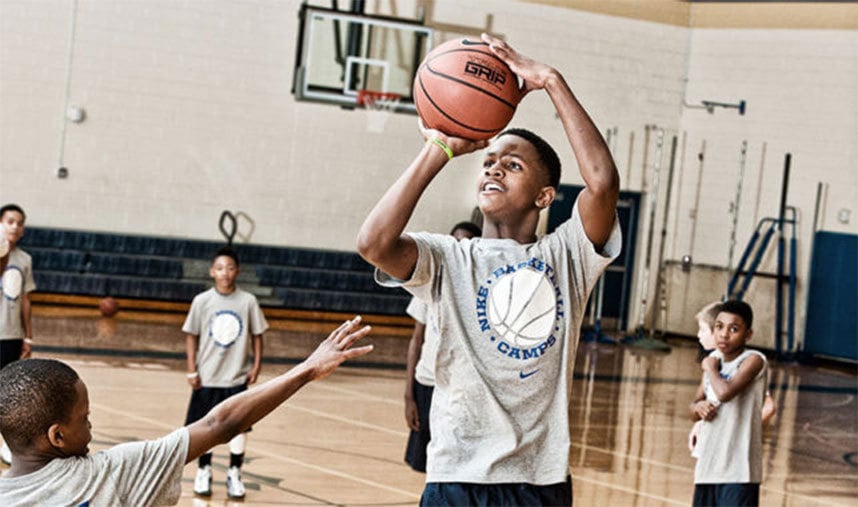The image captures a dynamic moment in a basketball game held in an indoor gymnasium. At the center of the scene is a young boy, likely around 13 or 14 years old, mid-jump with his hands raised above his head, gripping a basketball and looking determinedly towards the hoop, which is positioned off the photo to the left. He is smiling, seemingly anticipating a successful shot. The boy has black skin and is donned in a gray t-shirt emblazoned with the words "Nike Basketball Camps," featuring a basketball emblem in the center and the Nike logo beneath it.

To the left of the main player, another boy is actively trying to block the shot, with his arm outstretched in a defensive stance. Surrounding them are several other boys, younger in appearance—possibly nine or ten years old—all attentively watching the play unfold. The backdrop of the scene is defined by white brick walls and blue bleachers, with a visible gym mat in the right center area. The wooden floor is marked with various basketball court lines and symbols, adding to the authentic gymnasium atmosphere. Additionally, there is another basketball resting on the ground near the bleachers and some gym equipment scattered around. A basketball hoop is also visible in the background, indicating another potential play area within the gym.